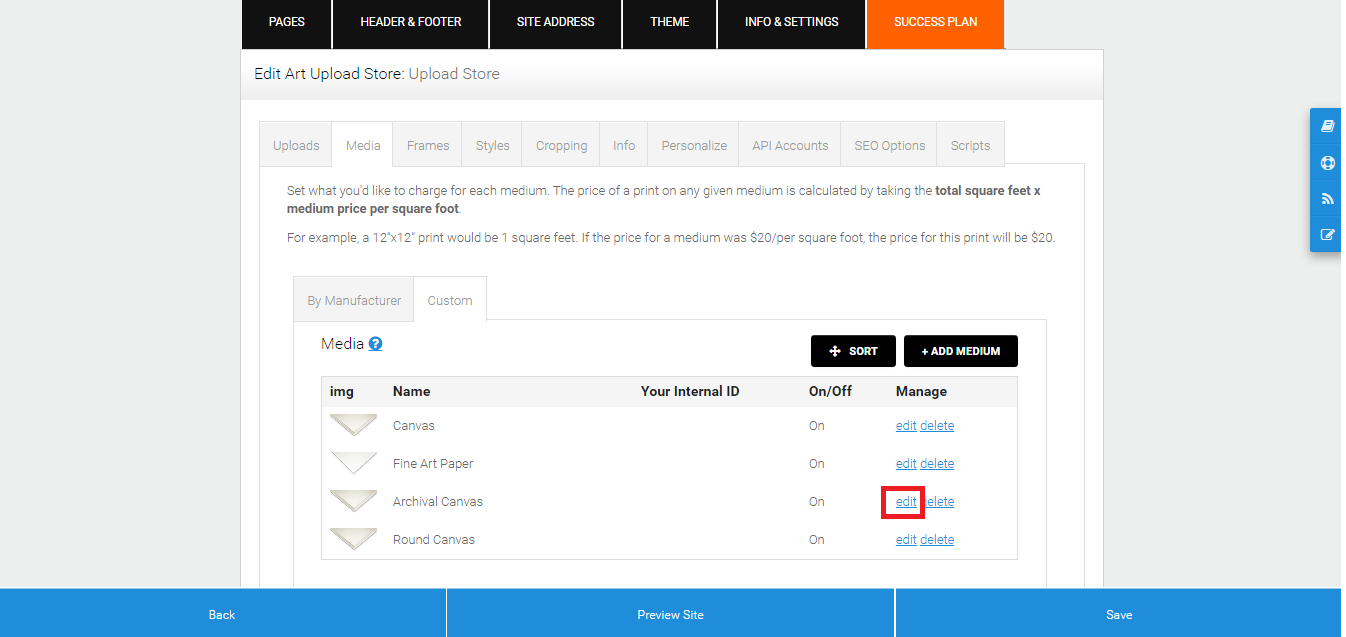Here is a detailed and cleaned-up caption for the image:

---

The image depicts a user interface for editing various settings on a web platform. The interface features two vertical gray borders on the left and right sides. At the top, there are different navigational sections labeled "Pages," "Header and Footer," "Site Address," "Theme," "Info and Settings," and "Success Plan." The "Success Plan" section stands out with an orange background and white font, while the other sections are in black with white font. 

Below these sections, on a gray and white background, are options labeled "Edit," "Art," "Upload," "Store," "Upload," and "Store." This is followed by a list of selectable options including "Media," "Frames," "Styles," "Cropping," "Info," "Personalize," "API Accounts," "SEO Options," and "Scripts," with the "Media" option currently selected.

Instructions are provided for pricing media, explaining that the cost of a print is determined by multiplying the total square feet by the price per square foot of the chosen medium. For example, a 12x12 print equals one square foot, and if the medium costs $20 per square foot, the print would cost $20.

The interface also shows media settings by manufacturer, with a "Custom" option selected. There are options to sort and add new media types, with available media including "Canvas," "Fine Art Paper," "Archaic Canvas," and "Round Canvas," all of which are turned on. On the right side, there are "Edit" and "Delete" buttons for each media type. One of the "Edit" buttons is highlighted with a red rectangle.

At the bottom of the interface, there are blue buttons labeled "Back," "Preview Site," and "Save."

---

This caption provides a clear and detailed description of the user interface, making it easy to understand the functionalities and options available.